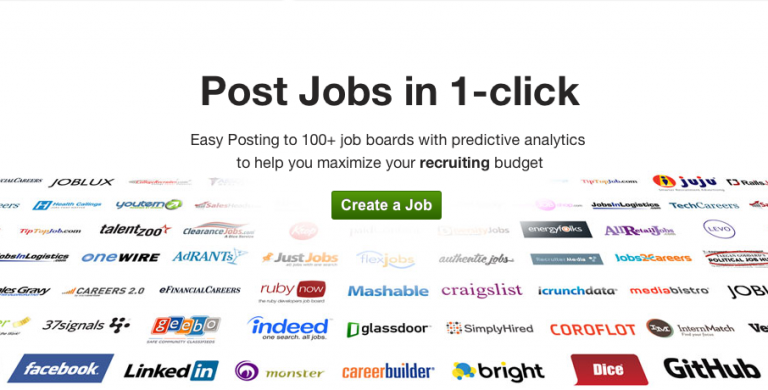This advertisement, set against a pristine white background, prominently displays the headline "Post Jobs in One Click" in large, bold black letters at the very top. Below, a detailed message in standard black font explains, "Easy posting to 100+ job boards with predictive analytics to help you maximize your recruiting budget," with the word "recruiting" emphasized in bold for extra impact. Directly below this text lies a vibrant green button inviting viewers to "Create a Job."

Occupying the lower half of the image and encircling the green button, there is a varied array of recognizable company and website icons. These icons showcase an impressive list of job boards and related services, including OneWire, Careers 2.0, 37signals, Facebook, AdRants, LinkedIn, JustJobs, Indeed, Monster, Mashable, Glassdoor, CareerBuilder, Craigslist, SimplyHired, Bright, ScrunchData, Coroflot, Dice, MediaBistro, and GitHub. At an angled perspective, making them slightly more challenging to discern but still present, are Joblox, Juju, and TechCareers, illustrating the extensive reach and comprehensive service offered by this job posting platform.